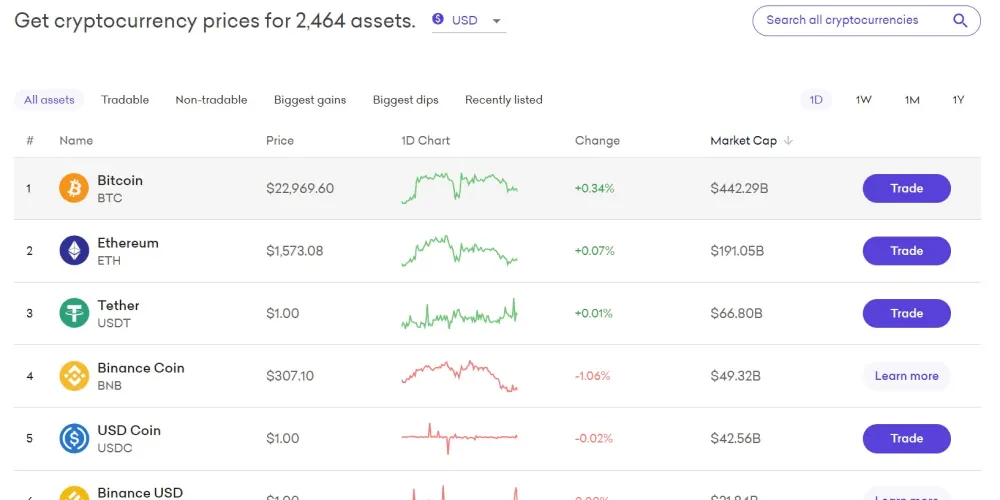This detailed screenshot displays cryptocurrency prices for 2,464 different assets, curated by a cryptocurrency specialist. It showcases a personalized portfolio including major cryptocurrencies like Bitcoin, Ethereum, Tether, Binance Coin, and USD Coin. The values of these shares demonstrate market volatility, with some experiencing a growth approximately of 0.34%, while others have declined in value. The fluctuating market prices are highlighted alongside the market cap for each asset. A distinctive feature is the purple text box labeled "TRADE" in white font, indicating the option for the individual to trade certain assets. The screenshot provides a dynamic view of the unpredictable nature of cryptocurrency investments.